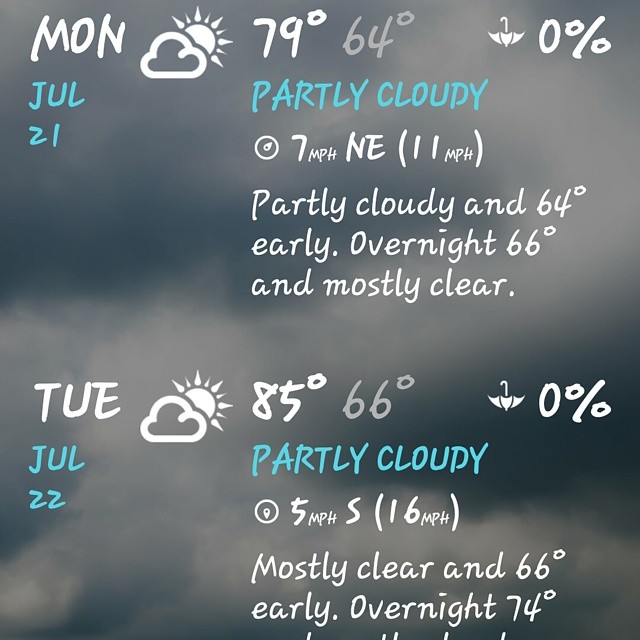The image is in portrait orientation with a blackboard-like background sprinkled with blotchy cloud patterns. At the top left corner, "Monday" is written in white, with an icon showing a sun partially obscured by clouds. Below, it indicates "79°F" as the daytime high and "64°F" as the evening low with a 0% chance of rain, symbolized by an upside-down umbrella. "July 21st" is written in teal, followed by "partly cloudy." The forecast continues with northeast winds at 7 mph, gusting up to 11 mph. It further states "partly cloudy and 64°F early," and "overnight 66°F and mostly clear."

Transitioning to Tuesday, identified as "July 22nd" in white text, the high is expected to reach "85°F" with a low of "66°F," again having a 0% chance of rain, depicted by another upside-down umbrella. The forecast mentions winds coming from the south at 5 mph, gusting up to 16 mph. The temperature is noted as "66°F early overnight" and climbing to "74°F." All text alternates between white and teal, providing a clear, detailed weather report over the next two days.